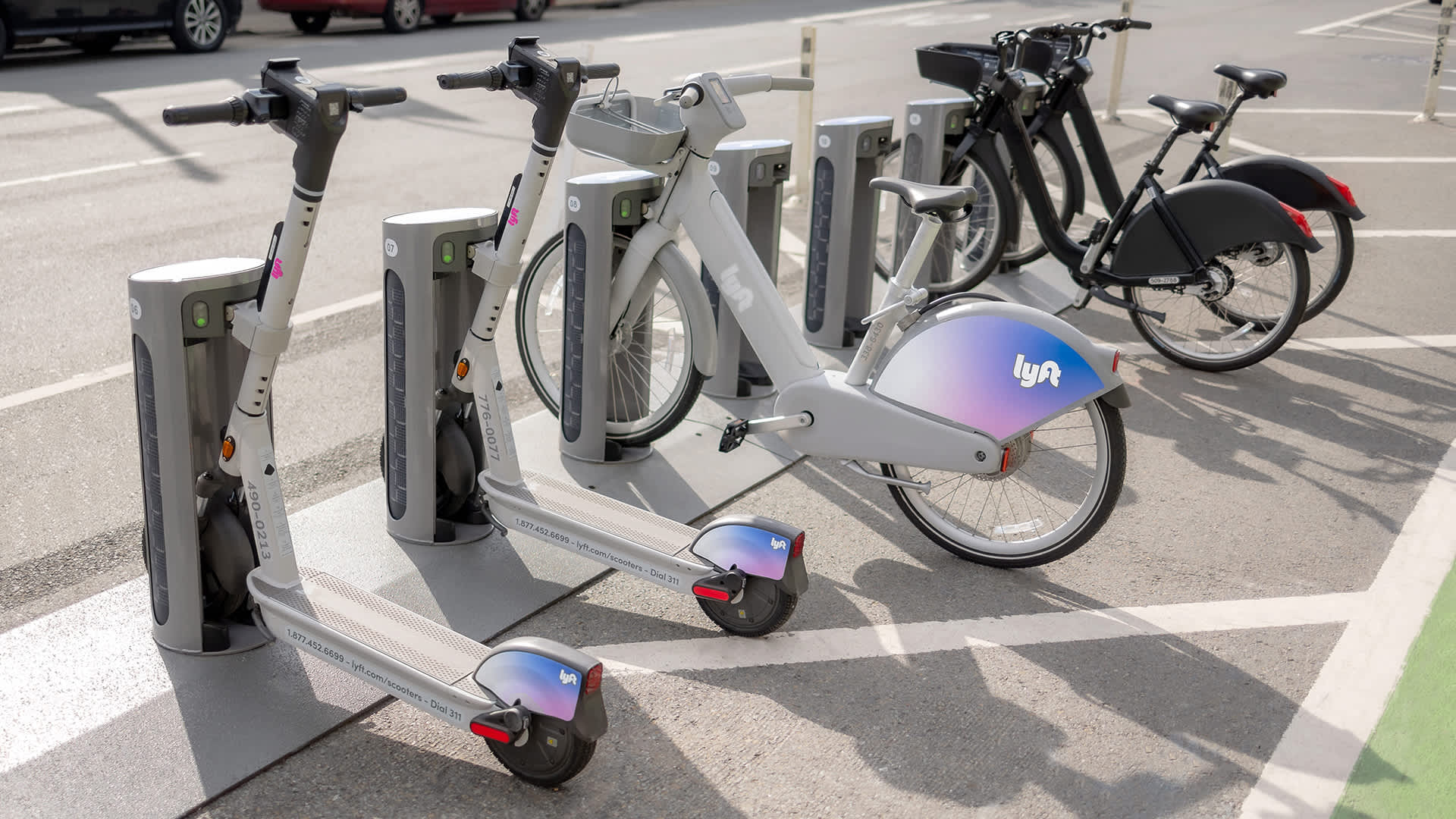This enhanced photo depicts a row of electrically charging Lyft scooters and bicycles, neatly arranged at a public rental port on the side of a street. The scene is captured on a sunny day, evident from the harsh shadows cast by the vehicles. The setup includes six, possibly seven, charging stations angled from the bottom left to the top right of the frame.

Starting from the left, the first two stations each harbor a white Lyft scooter, each featuring a gradient design transitioning from light gray to bluish-pink on the rear heel, along with the prominent Lyft logo. The third station houses a white Lyft bicycle, characterized by a front basket and a similar gradient design on the rear wheel cover, making it appear less realistic compared to the surrounding elements.

The next two charging stations are vacant, followed by two more stations that host nondescript black bicycles, each outfitted with front baskets and lacking any brand markings or advertisements on their all-black tires. A distinct feature of these bikes is the bright red light located at the rear, likely for nighttime visibility.

In the background, you can glimpse the lower parts of cars parked on the opposite side of the street, emphasizing the urban setting of this image.